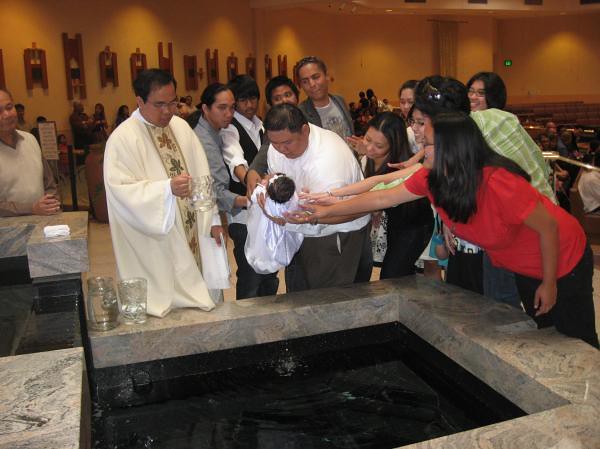The photograph captures a detailed and intimate moment of a child's christening or baptism set in a church. In the foreground, there is a stone baptismal font, rectangular and waist-high, filled with dark water shadowed from above. The font features a granite-colored counter and is flanked by two pitchers of water on the left side. Central to the image, a priest clad in tan-colored robes with white underrobes and a yellow floral patterned tabard is holding a half-filled pitcher. In a loving and solemn gesture, multiple family members, around ten in number, gather around as a slightly heavyset man in a white shirt and gray slacks holds an infant dressed in a silky, flowy gown over the font. Their hands are extended, either touching the baby or the man. Behind the group, the layout suggests a large congregation area with pews or possibly stadium-like seating, indicating a significant number of attendees witnessing the ceremony. The diverse group, primarily of Indian nationality, is unified in this sacred and celebratory act, with the communal act of blessing creating a profound sense of shared faith and tradition.